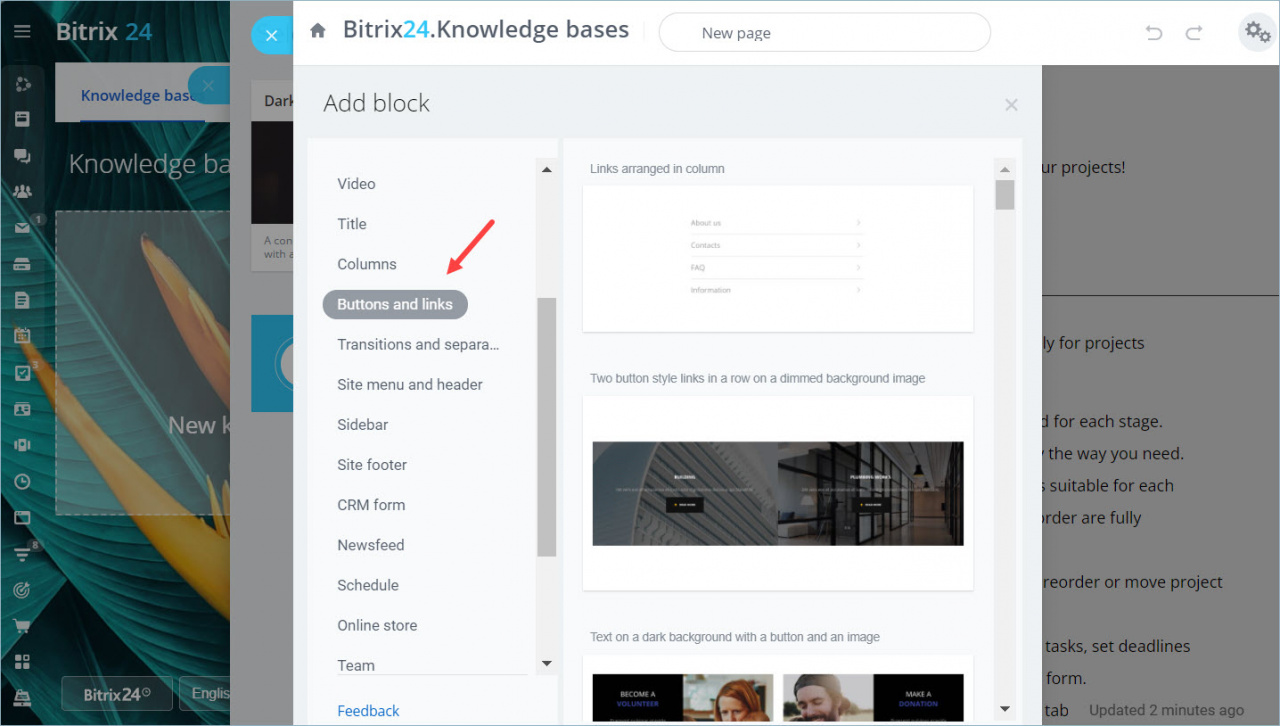The image showcases the user interface of the Bitrix24 website. The "Bitrix" part of the logo is displayed in white, while the "24" is in light blue. On the left-hand side of the screen, there is a shaded area with a bluish tint containing a vertical row of icons, partially obscured by a background image.

Adjacent to this shaded area is another section of the interface that appears greyed out, with a third overlay screen titled "Bitrix24.knowledgebases." This overlay includes various buttons, such as one labeled "New Page," and settings options represented by cogwheel icons on the far right.

Displayed prominently on this third screen is an "Add Block" title followed by a series of column options arranged vertically on the left. These options are labeled: Video, Title, Columns, Buttons and Links, Transitions and Separators, Site Menu and Headers, Sidebar, Site Footer, CRM Form, Use Feed, Schedule, Online Store, Team, and Feedback. The "Buttons and Links" option is currently selected and greyed out, indicated by a red arrow pointing to it. At the bottom, the "Feedback" option is a blue clickable hyperlink.

To the right of these options, a panel displays several images along with a section labeled "Links arranged in column," further detailing the interface's content and design layout.